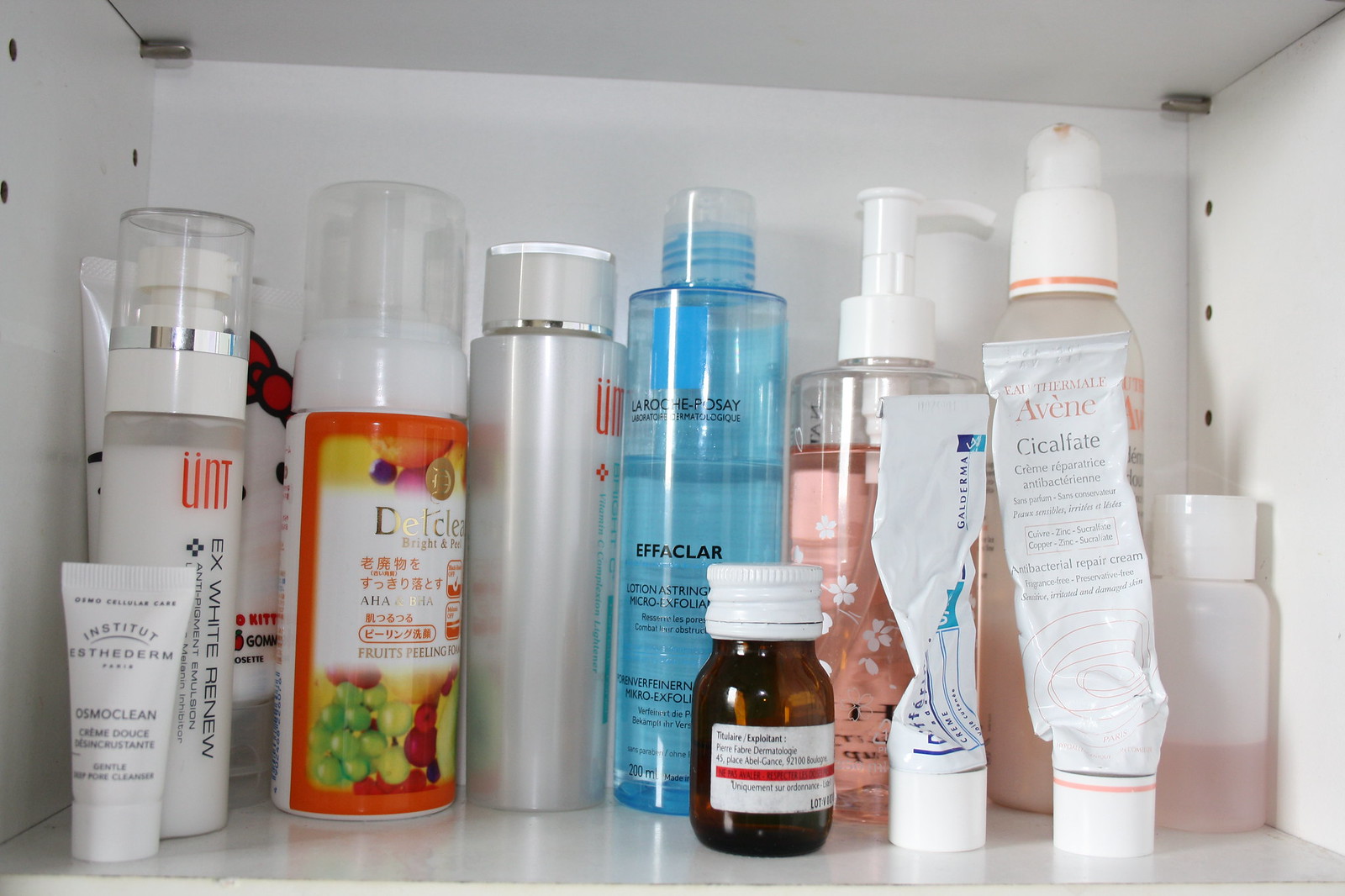An organized IKEA-style white medicine cabinet is open, revealing a neatly arranged collection of twelve beauty and skincare products on one shelf. The shelf is positioned with two inches of space above the items, allowing for easy access. 

From left to right, the collection begins with a small tube from the brand Institut Esthederm. Behind it, a white pump bottle from UNT labeled X-White Renew stands prominently. Next is a cheerful Hello Kitty-themed tube containing what appears to be bath gel. To its right is a pump bottle labeled in an Asian script, identified as Debt Clear with AHA, BHA, and fruit peeling serum. Following that is another container from UNT.

The next item is a clear plastic bottle filled with blue liquid from La Roche-Posay, specifically their Effaclar product. Positioned in front of the La Roche-Posay bottle is a tiny brown glass bottle with a twist-off metal cap, its label's text too small to read clearly. Adjacent to this is a well-used tube of what appears to be prescription skin medication.

Continuing, there's a clear plastic pump bottle containing pink liquid, likely soap. Right next to it is another pump bottle made of frosted clear plastic with a white top, though its label is unreadable. In front of this is a near-empty tube from Avène, known as Cicalfate. 

Lastly, on the rightmost side is a smaller white bottle with frosted plastic and a white cap, containing light pink liquid. The meticulous arrangement and varied product selection emphasize the careful curation of beauty and skincare essentials within this compact medicine cabinet.